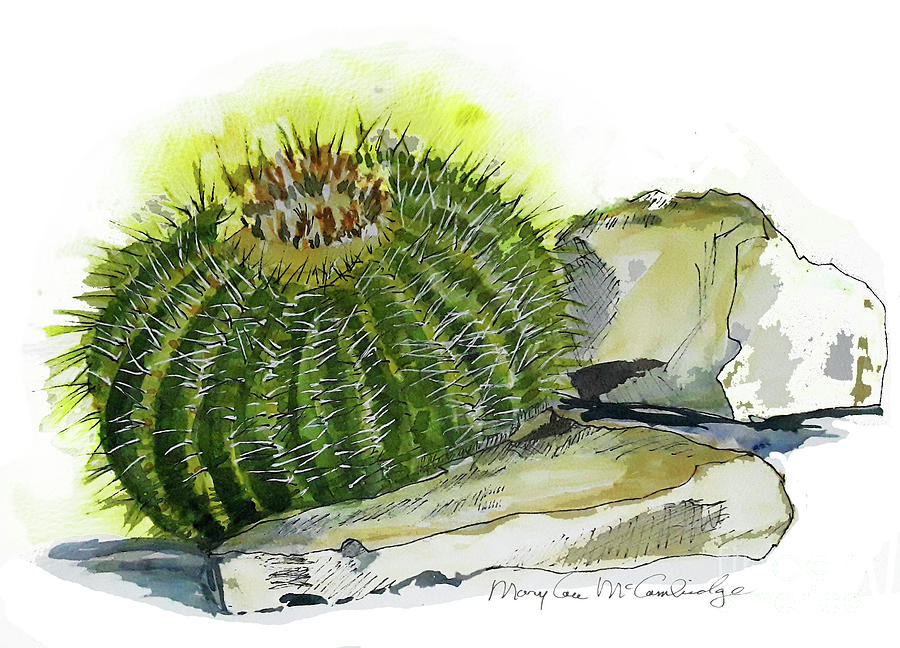This painting, signed by Mary Lou McCambridge, features a prominent, round barrel cactus depicted in rich green hues with gray-white needles. The top of the cactus showcases a distinctive reddish-brown flower or fruit. The artwork uses watercolor techniques, creating a soft emanation in the background, which is predominantly white with subtle shades of yellow suggesting a shadow on the wall. The cactus is nestled between two stones: one, a solid, flat slab situated in the foreground, and another, taller and triangular, positioned to the right. Both stones are rendered in shades of white, gray, yellow, and brown. The ground beneath them features nuanced tones of black and gray, emphasizing the overall earthy palette of the painting.